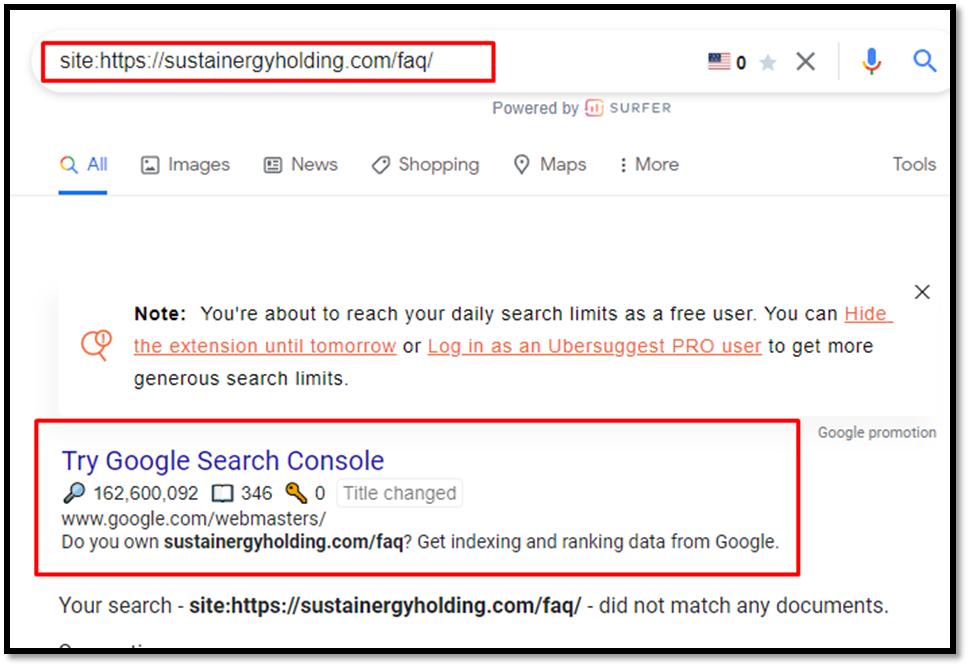A user is seen navigating Google with a sophisticated search query to gather information about Sustainergy Holding's FAQ page. They type into the address bar: `site:https://sustainergyholding.com/FAQ/`. The search engine promptly indicates that the user is nearing their daily search limit as a free user, suggesting they hide the extension or upgrade to UberSuggest Pro for more extensive results. Despite this, one of the top search results prompts the user to check Google Search Console for indexing and ranking data related to the sustainergyholding.com domain. This indicates the use of specific search operators to pinpoint precise information about the website. The result seems to suggest that the user might have ownership or administrative access to the site, or at least is interested in its performance metrics. Google, somewhat confused by the specificity of the query, presents results implying potential site ownership or managerial interest.